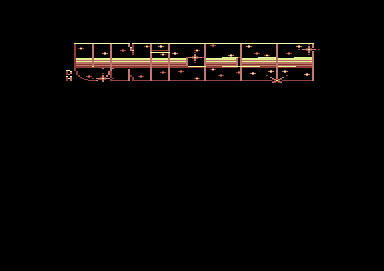The photograph presents a striking abstract image predominantly infused with bright yellows and deep blacks. Central to this picture is a complex composition that appears to spell out a word—possibly "union"—although its abstract rendering makes definitive interpretation challenging. This word-like structure is embellished with various characters and symbols, adding an enigmatic quality to it. Surrounding the letters are tiny gold dots, giving an impression of decorative stars, enhancing the overall visual intrigue.

At the top of the image, there's a long, thin rectangular box outlined in yellow, transitioning into orange on the sides, and culminating in brown vertical ends. Intriguingly, the interior of this rectangle is black, intersected vertically by several lines in a pattern: pairs of lines alternating with larger spaces. Smack in the middle of this black interior runs a yellow line flanked by multiple brown lines, some thin and some thick, contributing to a sense of division and structure.

Scattered throughout the image are small lights or dots of yellow with touches of brown, resembling tiny luminaries or decorative elements. The bottom left corner of the image features an amorphous shape that could be interpreted as a small character, reminiscent of pixelated figures from old video games, adding a nostalgic element. The high contrast between light and dark, coupled with meticulous detailing, creates an overall effect of dynamic abstraction, both difficult to decipher and richly intriguing.